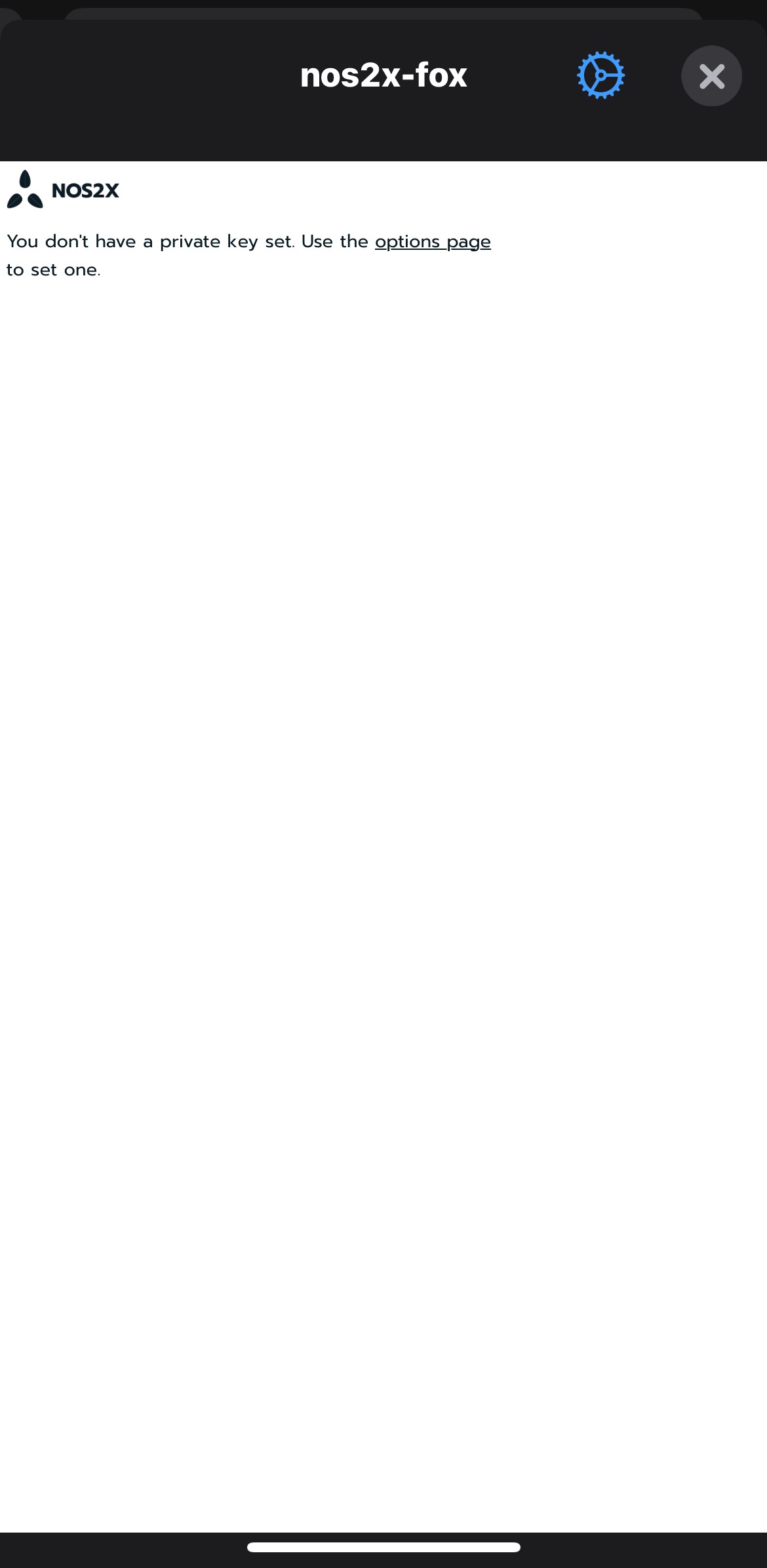A screenshot captures a mobile device interface, possibly from an Android or Apple device. Dominating the screen is a message indicating that "NOS2X-FOX" and a secondary entry, "NOS2X," are displayed prominently. The text mentions the lack of a private key setup, with a directive to visit the options page to configure one. The link to the options page is underlined, hinting at an interactive element for setting security parameters. The background of this alert is white, featuring small black text.

The "NOS2X" entry is accompanied by a distinctive icon resembling a triangle composed of three leaves at each corner, suggesting an emblematic or symbolic representation. At the top of the screen, a black bar with white text is visible, featuring a blue gear icon on the right, indicative of settings access, and an X button for exiting the current view. The overall impression is one of a security or encryption setup screen on a smartphone, with elements designed to facilitate user navigation and configuration.